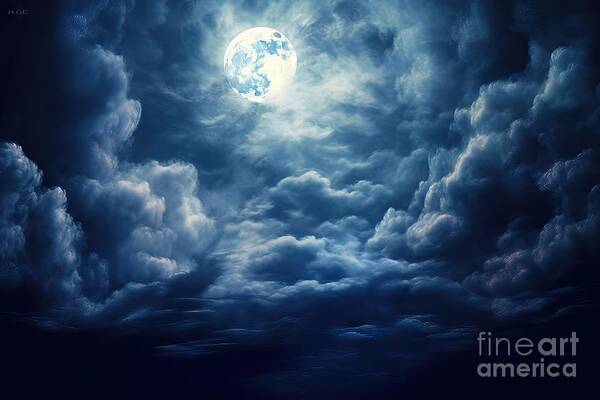This image from Fine Art America, with their logo in the bottom right corner, depicts a mesmerizing full moon in a moonlit sky. The moon, positioned slightly off-center to the left and near the top of the image, glows brightly, casting a blue light that illuminates the surrounding clouds. The darker areas on the moon appear in shades of blue, resembling continents, adding a surreal quality to its appearance. Thick, puffy clouds roil around the moon, with those closest to it glowing whiter and shinier due to the intense lunar light, while the clouds at the edges of the image darken to deep blue and gray hues. The overall composition gives the impression of the moon nestled within a cave or womb of clouds, creating a scene with significant depth and an almost otherworldly atmosphere.